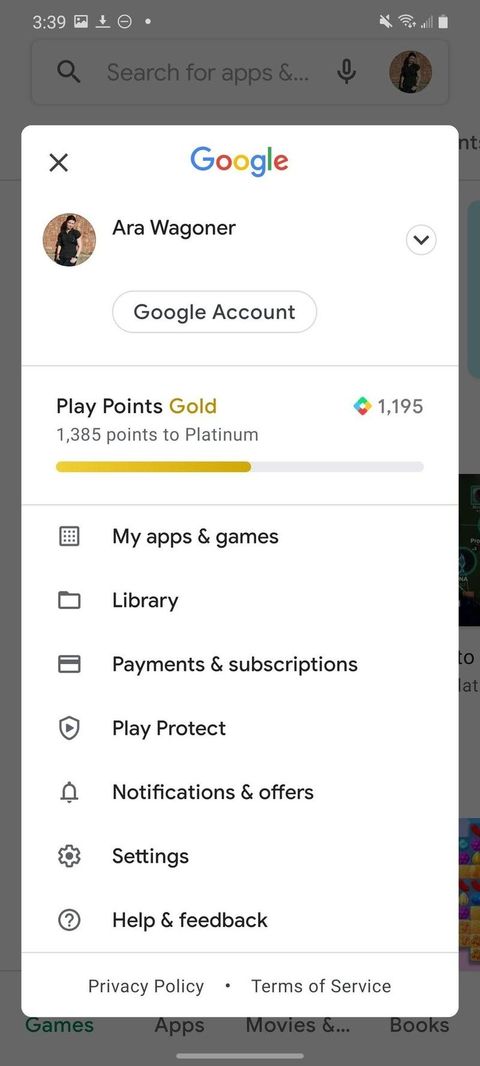Screenshot of Smartphone Google Account Pop-up at 3:39 PM

In this detailed screenshot of a smartphone, the status bar at the top displays the current time, 3:39 PM, in the upper left corner. To the right of the time, four icons are visible in white font: the sound icon, the Wi-Fi signal icon, the cell signal icon, and the battery life indicator.

The main focus of the screenshot is a prominent Google pop-up window. At the top of this window is the Google logo, with an 'X' button to the far left corner for closing the pop-up. Below the logo, there is a user account section featuring a circular photograph on the left, presumably of the user's profile picture, labeled "Ara Wagoner." To the right of the name, there is a downward arrow indicating a drop-down menu.

Immediately beneath this section, a white button labeled "Google Account" in black font is placed. A thin gray line divides this part from the next section below.

The next section displays "Play Points Gold," with the word "Gold" highlighted in gold font. It indicates "13.85 points to platinum" and shows the current balance of points as "11.95." Adjacent to this is a horizontal progress bar that is about halfway filled, with the filled portion also in gold.

A second gray line separates this section from the final part, which lists several selectable options such as My Apps and Games, Library, Payments and Subscriptions, Play Protect, Notifications and Offers, Settings, and Help and Feedback. Each option is paired with a small icon and rendered in black font.

At the very bottom of the pop-up window are links to the Privacy Policy and the Terms of Service, separated by a centered dot.